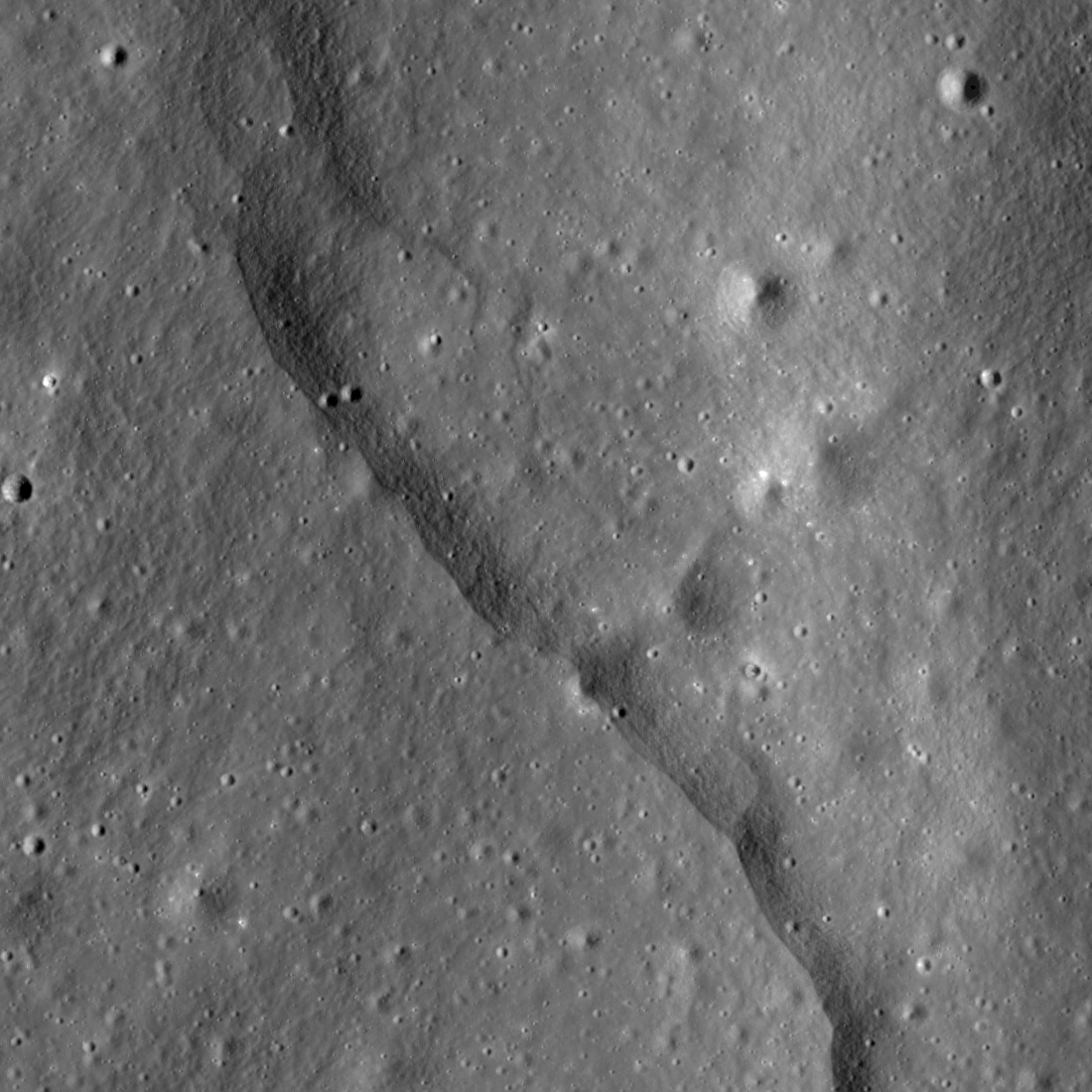This black and white aerial photograph, likely taken by an esteemed professional, showcases the surface of the Moon from orbit. The square image reveals an uneven, texturized expanse resembling a gray skin dotted with small craters, much like tiny bumps or pimples. There are a few moderately larger craters scattered across the surface, with notable ones positioned on the left, upper right, center, top, and bottom. A distinctive raised ridge or fissure runs diagonally from the lower right to the upper left corner, cutting through lighter and darker patches of the terrain and suggesting a dynamic lunar landscape. The overall appearance gives a close-up, detailed view of the Moon's rugged and cratered surface.